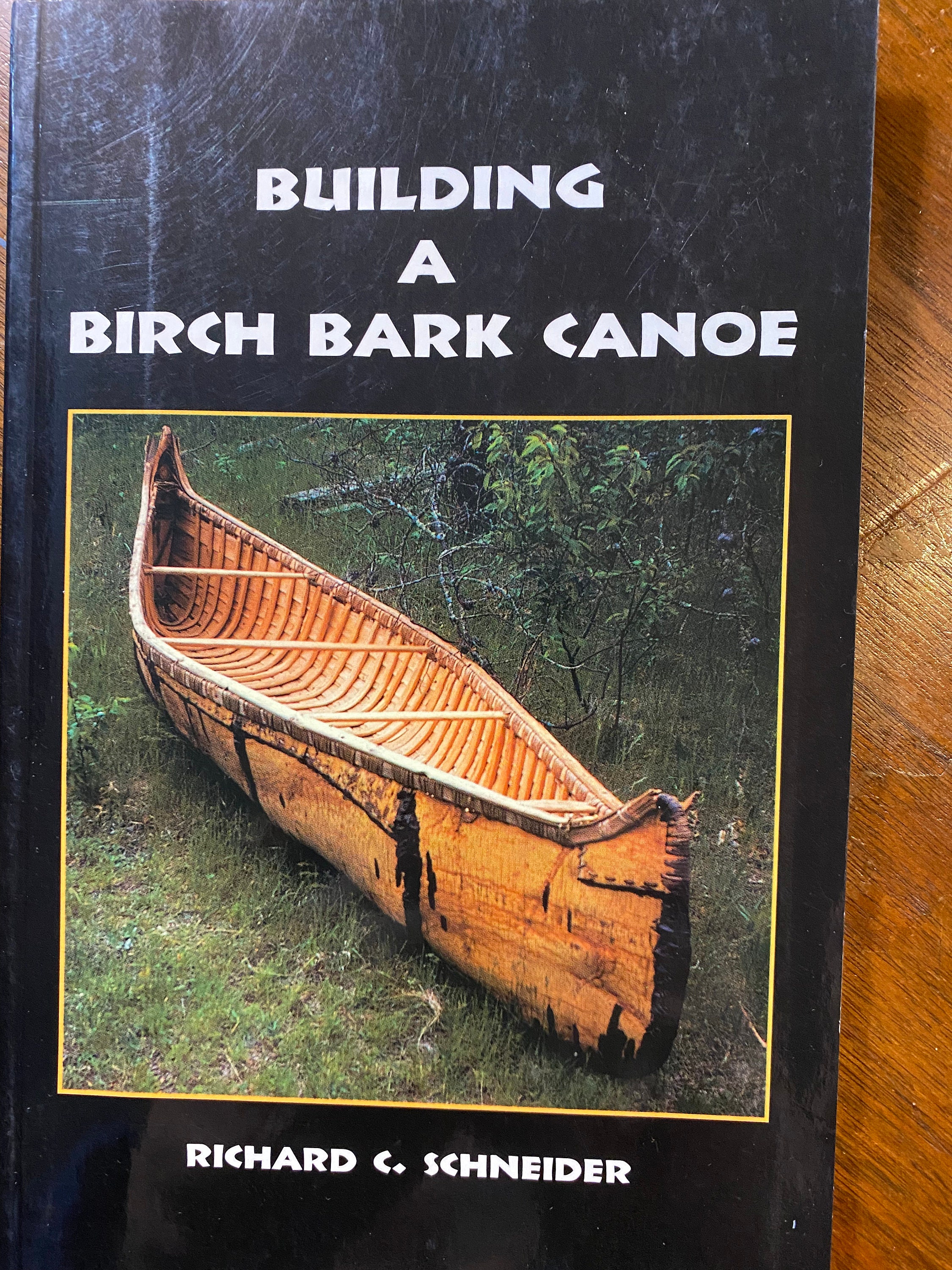A hardcover book titled "Building a Birch Bark Canoe" by Richard C. Schneider is laid out on a dark brown wooden table. The black cover of the book, scratched and worn, showcases a central square image with a light yellow border. The image depicts an old wooden canoe, characterized by its medium brown color and some black areas along the edges. The canoe, with raised arc sections inside and three planks crossing the top, is set against a green grassy background, surrounded by small plants and trees. The title and author’s name are prominently displayed in white, all-caps text, positioned at the top and bottom of the cover respectively.